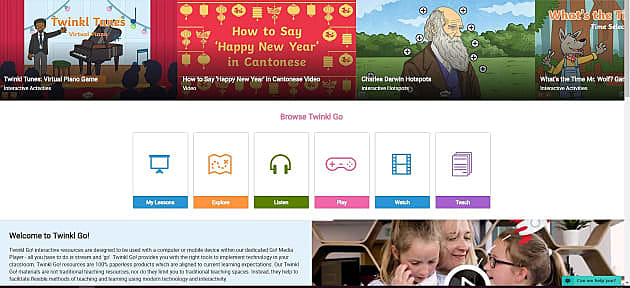This image is a low-resolution screenshot of a website, making some of the text difficult to read due to its blurriness. The rectangular image is structured like a gallery of articles at the top. 

On the left side, there's an illustration of a man standing on a stage next to a piano, framed by red curtains. Next to this is a red box containing text in yellow that says, "How to say Happy New Year in Cantonese," surrounded by Chinese lanterns.

To the right of this, there's an illustrated picture of Charles Darwin accompanied by numerous plus signs. Further to the right, a cartoon dog wearing a long-sleeved yellow shirt and blue overalls stands in front of several brown tree trunks.

Below these images, large text reads "Browse Twinkle Go," followed by a series of boxes featuring different icons and colors, including a blue projector screen, orange map, green headphones, pink console, blue film reel, and purple papers.

At the bottom, a blue box welcomes users with the text "Welcome to Twinkle Go," and on the right-hand side of the screen, there's a small video featuring a mother with two children.